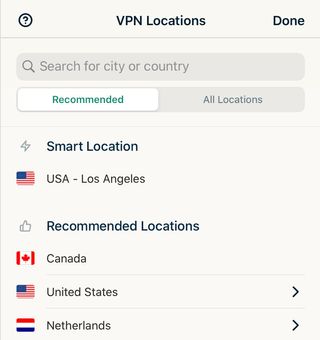The image is a detailed list of VPN locations presented in a square format with a subtle off-white background. 

In the upper left-hand corner, there is a question mark enclosed in a circle, likely indicating a help or information feature. At the center top, the title "VPN Locations" is prominently displayed, while the upper right corner features a "Done" button. These elements are separated from the main list by a horizontal gray line.

Below the line, there is a darker gray search bar that prompts the user to "Search for city or country," allowing easy navigation through the VPN options.

The list begins with a section titled "Recommended," highlighted in green font within a white button. To the right of this section is another tab labeled "All Locations." Another horizontal line divides this part from the detailed list of VPN options.

The first entry is under the heading "Smart Location," suggesting the best server choice, which is "USA Los Angeles." This entry is complemented by the American flag icon.

Below the smart location, the "Recommended Locations" section lists:
1. Canada, marked with the Canadian flag.
2. United States, accompanied by the American flag.
3. Netherlands, signified by the red, white, and blue stripes of the Dutch flag.

Each recommended location features a thumbs-up icon to the left, indicating approval or suitability.

This chart is designed to help users select their preferred VPN location and seamlessly continue their internet activities.